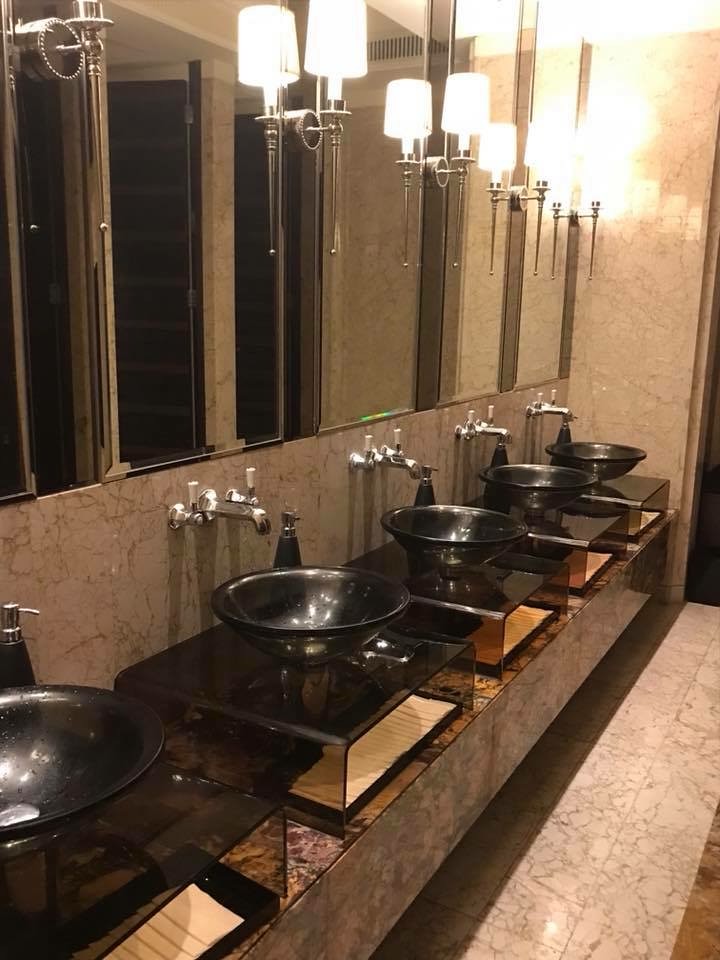The photograph captures an elegantly designed public bathroom, with a side-angle view emphasizing a row of five sleek, black bowl sinks mounted on dark, smoked glass pedestals. The sinks are complemented by chrome spigots with vertically oriented white porcelain handles emerging from a textured tan marble wall, which features intricate brown cracks giving it a rugged appearance. Each sink is paired with a tall, rectangular mirror adorned with attached light sconces. These sconces, crafted from polished steel or chrome, hold single candle-shaped lamps encased in cylindrical shades, casting a warm glow that highlights the clean, modern aesthetic. Below each sink, a neatly folded hand towel or possibly soap rests on the shelf, adding to the bathroom's refined functionality. The floor consists of light tan tiles with darker veins, enhancing the textured theme, while additional elements, such as black soap dispensers with silver tops, complete the sophisticated look of this well-appointed lavatory space.